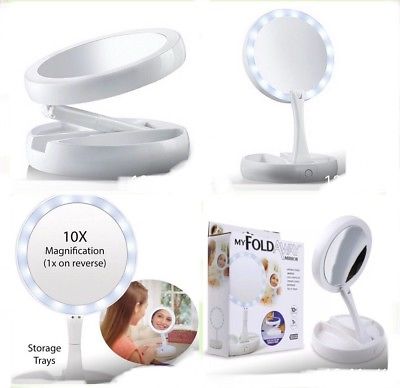Here is a cleaned-up, detailed caption for the image:

---

The image features a compact, white collapsible face mirror, showcased against a white background in four distinct sections. In the upper left corner, the mirror is displayed in its collapsed state, illustrating its portable, suitcase-friendly design. To the right of this, the mirror is shown unfolded and upright, highlighting its built-in LED lights that encircle the mirror, providing illumination ideal for detailed facial care such as pore inspection.

In the lower right corner, the same upright mirror with its LED lights on is depicted, with text written inside the mirror indicating "10x magnification, 1x on the reverse." At the base of the mirror image, the phrase "storage trays" is noted, emphasizing the additional feature of the mirror’s base.

In the lower left corner, there is a photograph of the product’s cardboard packaging. The packaging is primarily white, with "MyFold" emblazoned in black font at the top. Below this branding is an image of the same illuminated upright mirror.

---